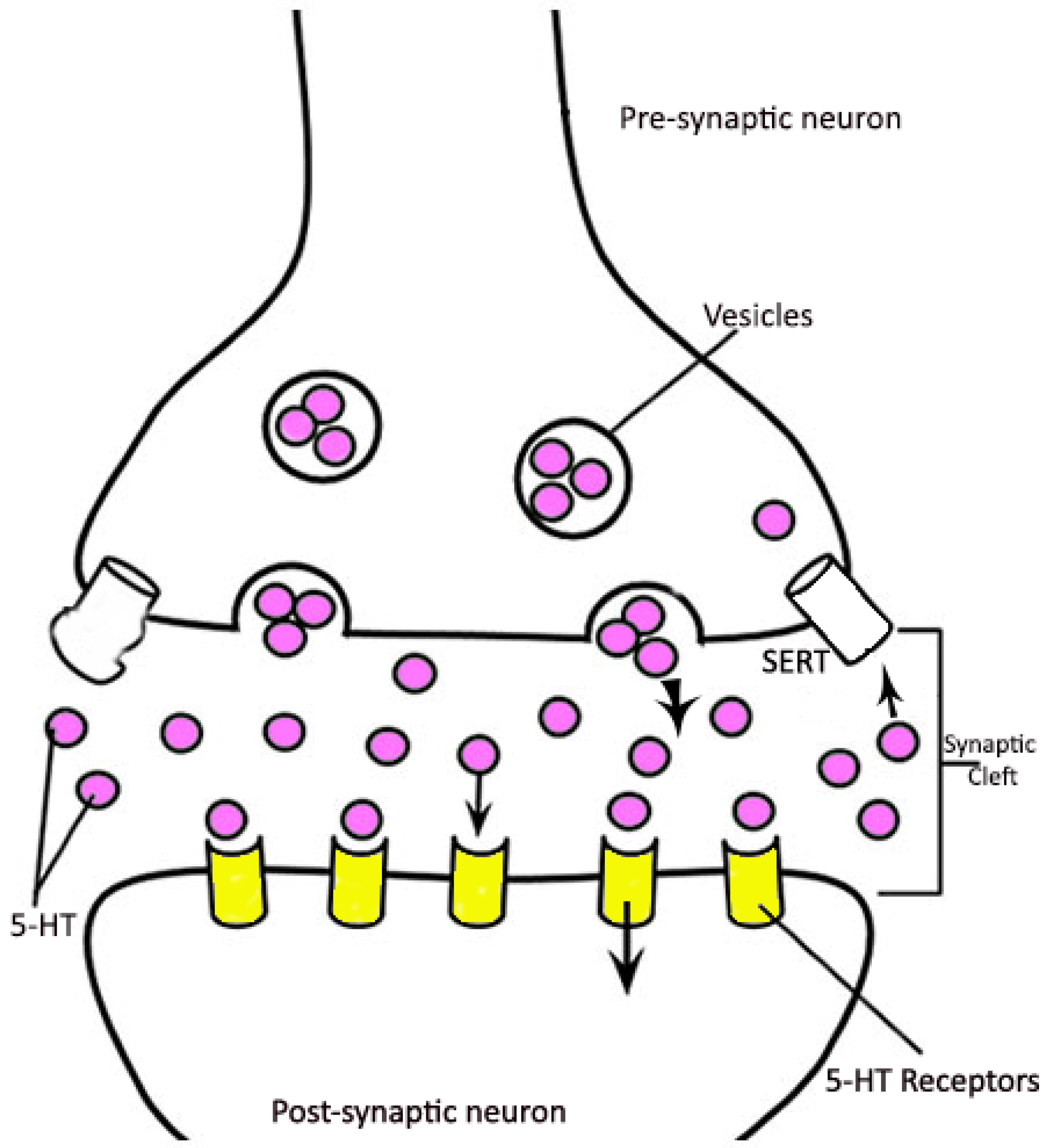This scientific drawing is a detailed illustration of the synaptic process between neurons, focusing on the transmission of 5-HT (serotonin) from the presynaptic to the postsynaptic neuron. The image predominantly uses black, white, pink, and yellow colors. At the top, the presynaptic neuron is labeled and contains vesicles, which are clusters of pink or purple dots. These vesicles encompass multiple 5-HT molecules, indicated by red or pink circles labeled "5-HT." The presynaptic neuron releases these vesicles into the synaptic cleft, the space between the two neurons.

Within the synaptic cleft, which is clearly labeled, the 5-HT molecules are visible as scattered pink dots. There are several black arrows in the diagram, indicating the direction of movement of these molecules. The bottom part of the illustration features the postsynaptic neuron, marked with yellow cylindrical shapes that represent the 5-HT receptors, responsible for receiving the serotonin. Additionally, the diagram includes the term "SERT" on a white cylinder, which likely refers to the serotonin transporter involved in reuptake. The entire image is annotated with labels like “presynaptic neuron,” “vesicles,” “synaptic cleft,” “5-HT receptors,” and “postsynaptic neuron,” providing a comprehensive view of the synaptic transmission process.